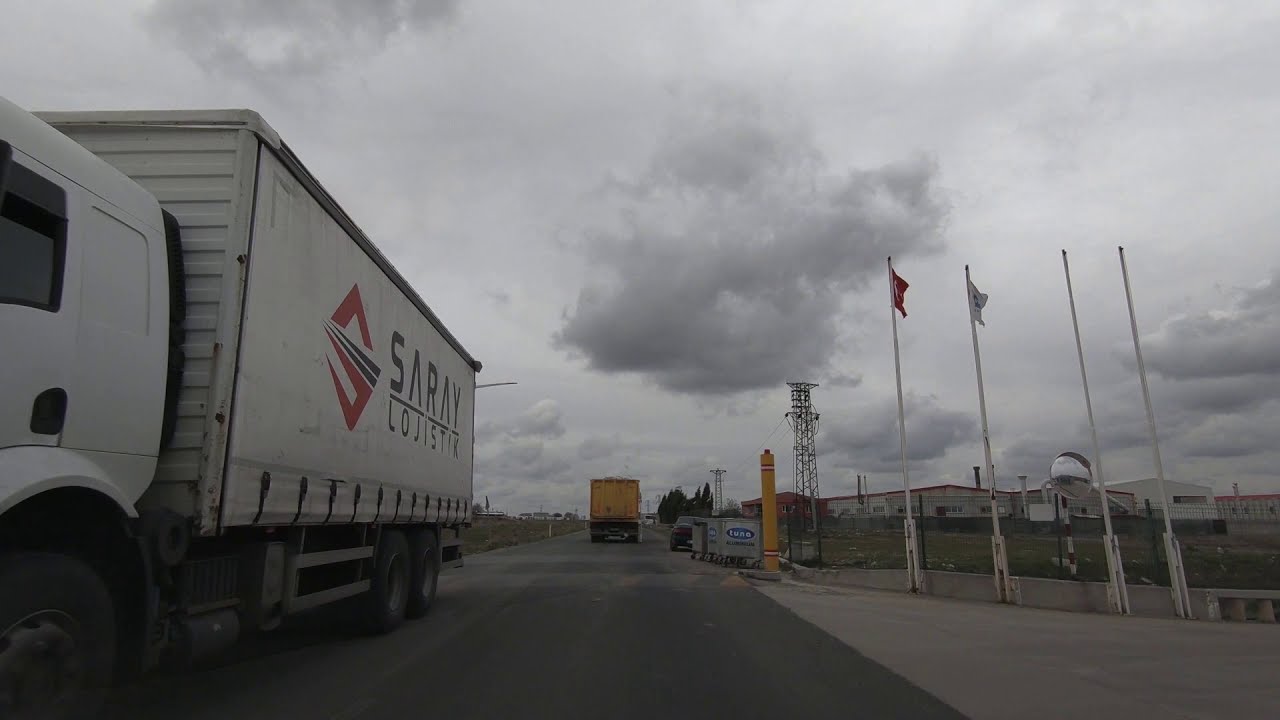This photograph captures a bustling distribution center under an overcast sky filled with dark gray clouds. The main focus is on a large white semi-tractor trailer on the left side of the image, moving towards the camera and nearly out of frame. The side of the truck prominently displays the company's name "Saray Logistics," spelled out in black letters with a red and blue logo beside it. Beneath the main text, "Logistik" is written in a similarly stylized font. In the center of the image, a blacktop road extends from the bottom center towards the horizon, guiding the viewer's eye deeper into the scene.

Further down the road, a yellow truck is seen heading north, while smaller trucks are also traveling in the same direction, contributing to the sense of activity. Four flagpoles on the right side of the photograph add a touch of verticality, while beyond them, industrial buildings and telecommunication antennas rise within a fenced area. A small cart with the word "Tuna" displayed in white text on a blue background can be spotted near the center of the image, adding a detail that hints at the variety of goods distributed here. The photograph paints a vivid picture of a busy logistics hub with its blend of moving vehicles, infrastructure, and indefinable flags fluttering under a moody, gray sky.